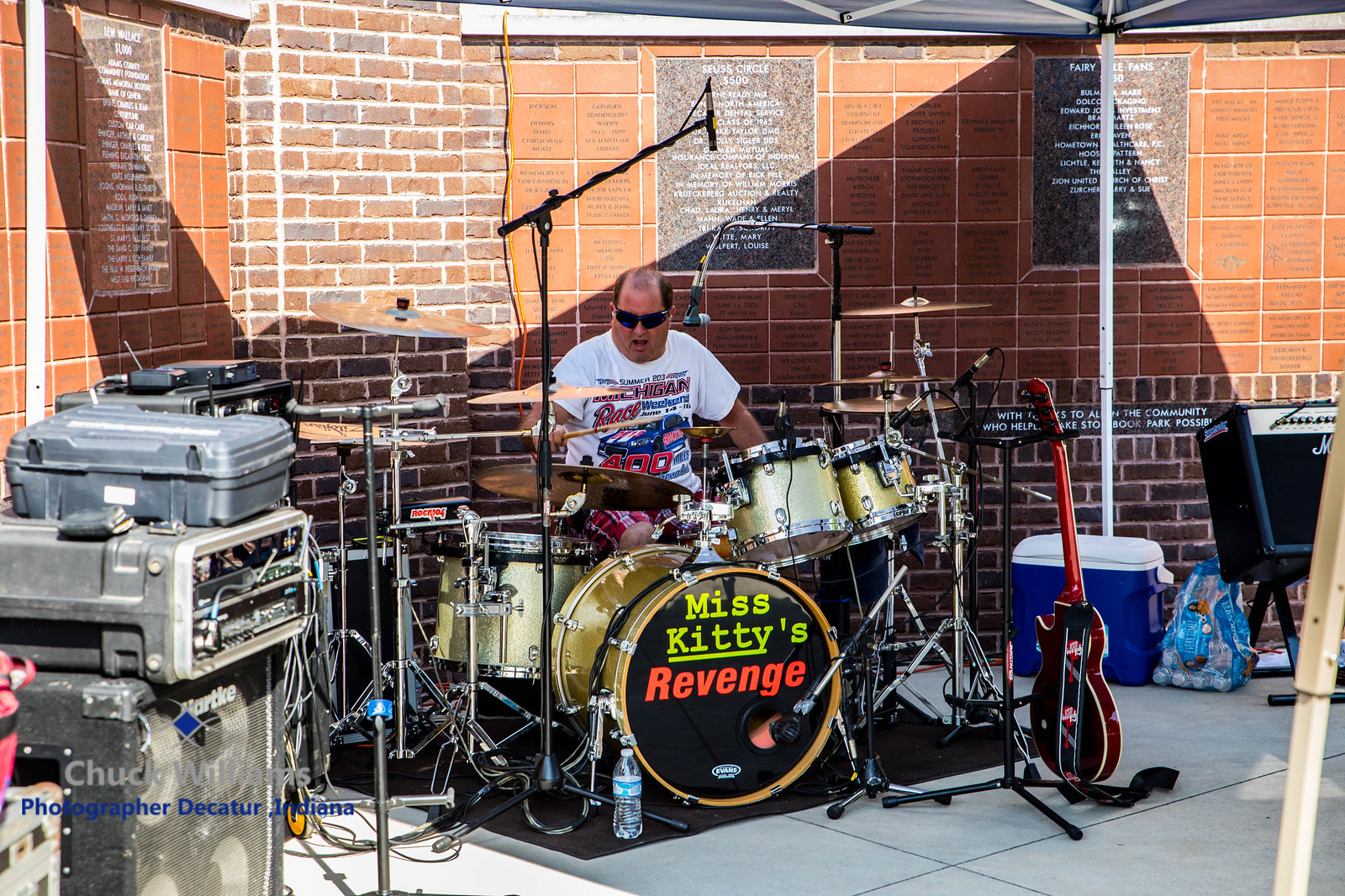In this vibrant outdoor scene, a balding, middle-aged man in a white t-shirt featuring a "Michigan Race" graphic is intensely playing a large, sparkling gold drum set. The setup is under a pop-up tent on a concrete pad, providing shade from the bright sunny day. Surrounding him are various pieces of music and electronic equipment, including a guitar on a stand and a blue cooler filled with water bottles. Multiple microphones are strategically placed around the drum set, including one close to his face to capture his every move. The prominent bass drum proudly displays the text "Miss Kitty's Revenge." Behind him, a brick and red tile wall, adorned with names and sayings that resemble a memorial, serves as the backdrop. A photo credit at the bottom left corner reads "Chuck Williams, photographer, Decatur, Indiana."